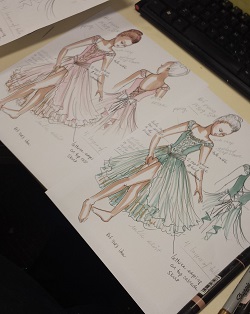The image showcases detailed sketches of two ballerinas on white paper, angled against a black surface. Each ballerina is depicted in both front and back views in elaborate dresses, with one set being pink and the other green. Both designs are similar, featuring corseted backs. The sketches include various notes, arrows, and detailing across the illustrations. One ballerina has white hair while the other has reddish-brown hair, each in a graceful dance position with legs crossed and arms poised. Next to the drawings, there are black and gray pins. The drawings are executed in brown and green hues, suggesting an emphasis on design elements and structure of the ballerina dresses.